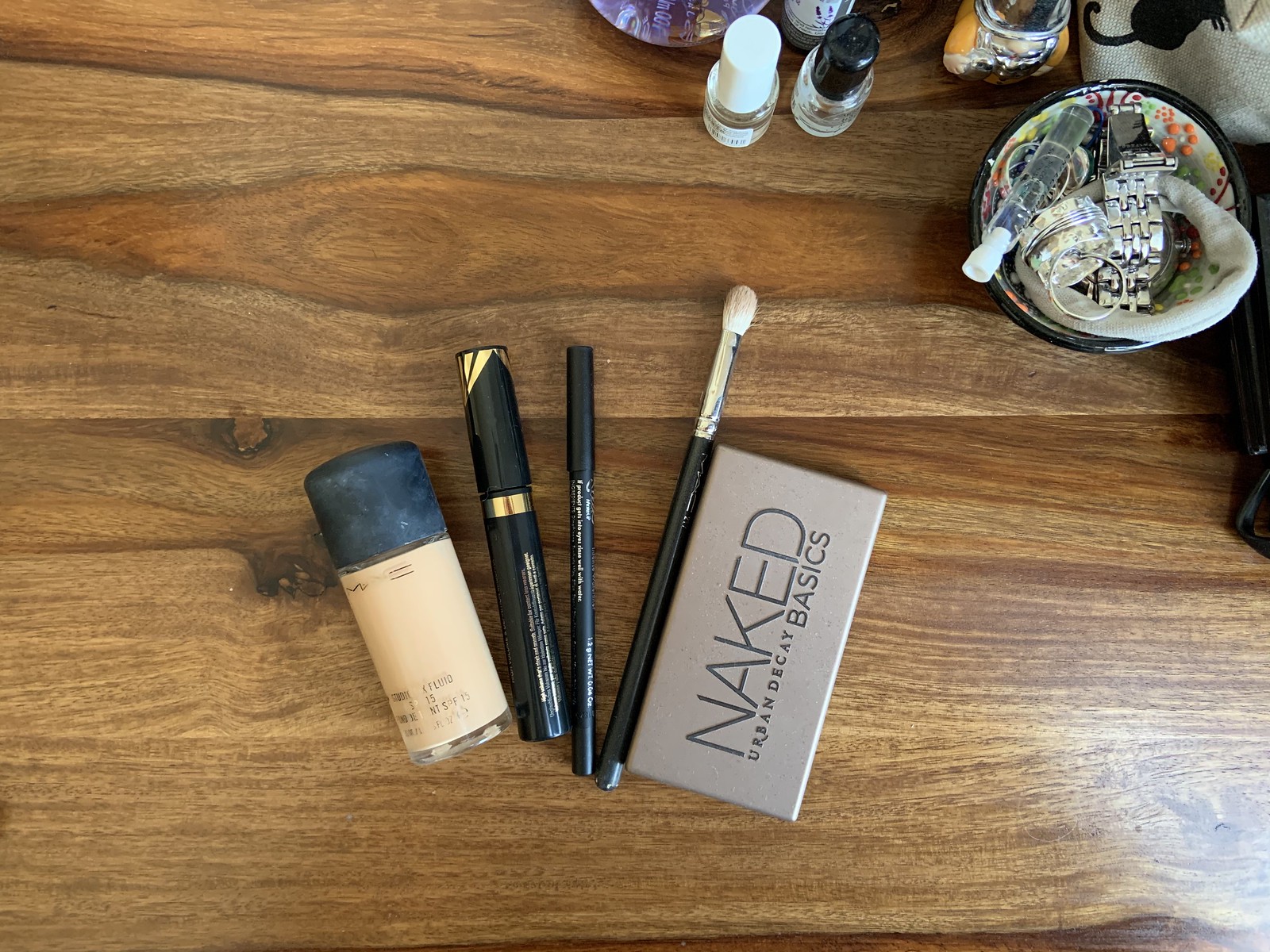This photograph captures an assortment of cosmetic and personal care items carefully arranged on a richly textured wooden table. The table itself features a striking mix of orangey, light, and mid-tone wood grains, with a slightly reflective surface showing light gouges and marks that add character. 

Prominently centered is a bottle of MAC foundation in a light skin tone shade, capped with a sleek black lid. Nearby, a sophisticated black and gold wand stands upright next to a slender black makeup item adorned with delicate gold font. A black, silver, and white makeup brush lies adjacent to a "Naked Urban Decay Basics" palette, which has a tan cover with darker lettering.

In the background, a black ceramic dish with a vibrant, colorful pattern holds a silver wristwatch and a few miscellaneous items. Two bottles, one clear with a black lid and another white with a white lid, are placed on the table. A fabric item depicting a black cat adds a whimsical touch, while various other miscellaneous objects subtly clutter the background, completing the scene.